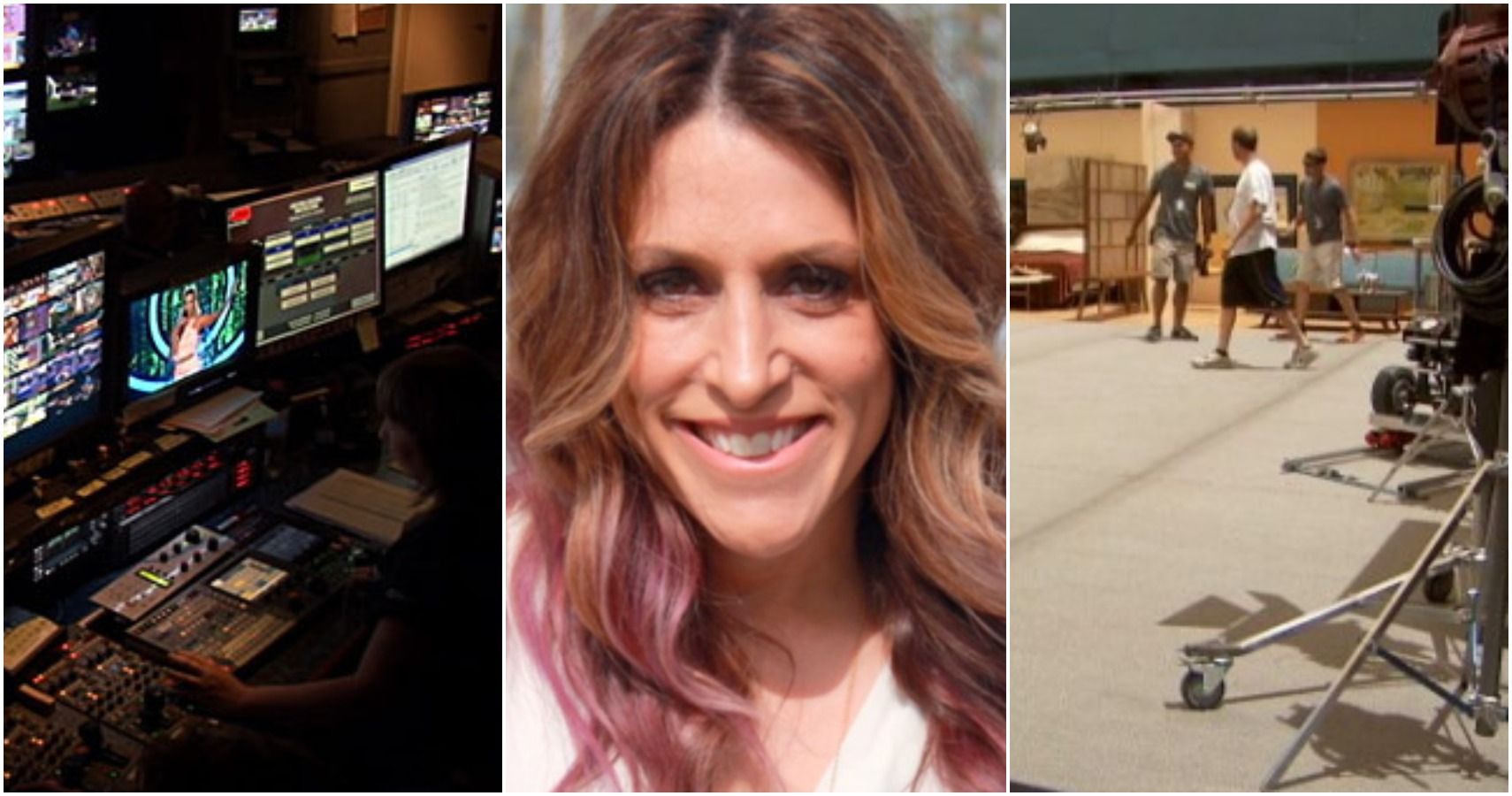This collage image is divided into three equal thirds. 

On the left, we see a detailed control room, potentially a recording studio for television, filled with numerous monitors, switchboards, and sound equipment. A person, possibly a female, is seated at a desk, engaging with the control panel and gazing at the monitors. The image captures her from a side view, emphasizing her left arm poised to press several buttons.

The central image features a close-up of a smiling woman with long, wavy brown hair accented with pink highlights and platinum streaks towards the bottom. She is wearing a white shirt and appears to be in her mid-30s. Only her face, neck, and the upper part of her torso are visible.

The right third of the collage depicts three men walking through a large, open room with tan flooring. Two wear gray shirts, and one is in a white shirt, engaged in conversation. This setting appears to be part of a studio or a set, with some visible metallic equipment legs suggesting a workspace for assembling or adjusting the studio set.